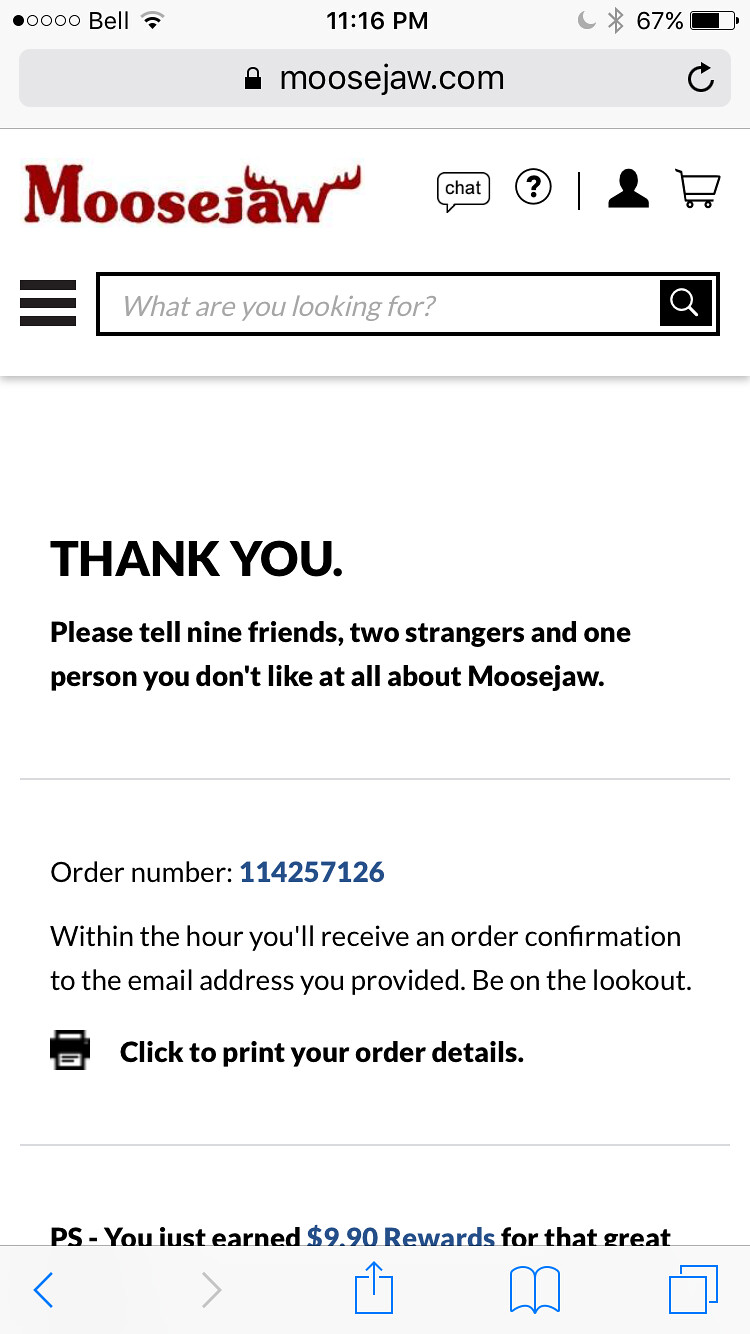The image depicts a screenshot from a mobile browser displaying an order confirmation webpage from Moosejaw.com. At the top, the connectivity indicators show it’s 11:16 PM, with Bell service, WiFi, Bluetooth connected, and 67% battery life. The web address bar shows "moosejaw.com." Prominently featured is the Moosejaw logo in red with antlers sprouting from the "W." The site includes icons for chat, help, account, shopping cart, and a search bar reading "What are you looking for?"

The central message, in bold black capital letters, reads: "THANK YOU! Please tell nine friends, two strangers, and one person you don’t like at all about Moosejaw." Below this, an order number 114257126 is displayed in blue. Additional text informs the viewer that an order confirmation will be sent to their email within the hour, with a note about having earned $9.90 in rewards. There is a printer icon for printing order details. The overall style underscores a modern e-commerce interface with humorous, engaging text aimed at encouraging word-of-mouth promotion.